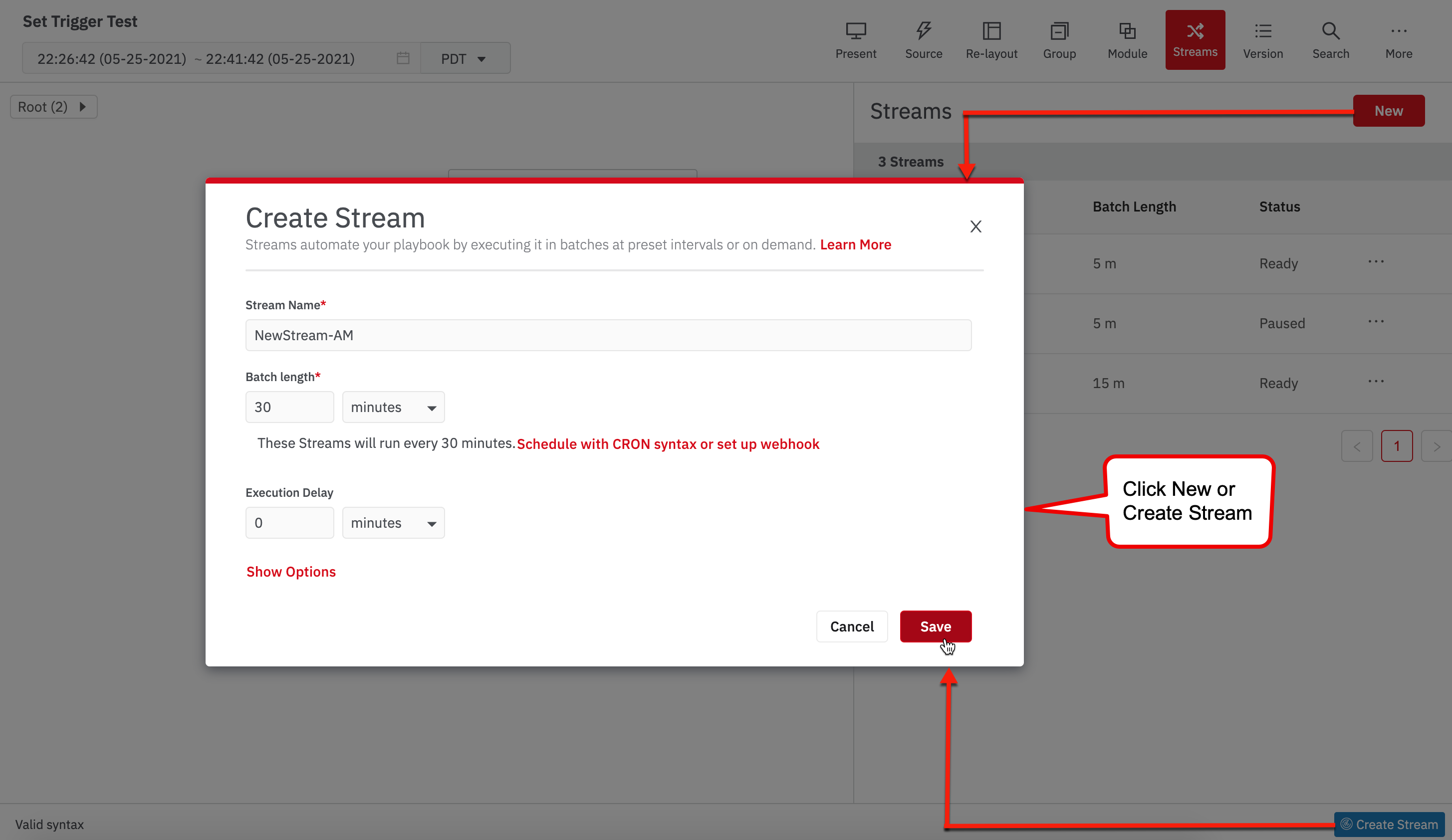The image features a gray background with several interface elements prominently displayed. At the top, there is a section labeled "Set Trigger Test," followed by buttons and tabs such as "Present," "Source," "Relay Out," "Group," and "Module." A red square highlights one of these tabs, and alongside is the "Version Search" option and a menu symbolized by three horizontal dots.

In the middle of the interface, there is a red rectangle labeled "New" with white text, alongside a blue rectangle labeled "Create Stream," also with white text. A red arrow pointing upwards connects "Create Stream" to a white box, while another red arrow pointing downwards links "New" to a different white box.

The upper white box features a red header labeled "Create Stream," includes some unspecified information, and has a clickable "Learn More" in red. This box also includes a "Close" button marked with an 'X,' a "Stream Name" field indicated by a red asterisk, a text box for input, and another field labeled "New Stream."

Further details within the interface include a section titled "Batch Length," where the default value is '30' and units are specified as minutes. A note beside it explains that these streams run every 30 minutes. There is also a red-labeled "Schedule" section, which uses CRON syntax or can be set up as a webhook.

Another part of the interface is the "Execution Delay" feature, which includes two input rectangles, one labeled '0' and the other 'Minutes.' A red "Show Options" link provides additional configuration choices.

On the right side, the interface lists three active streams.